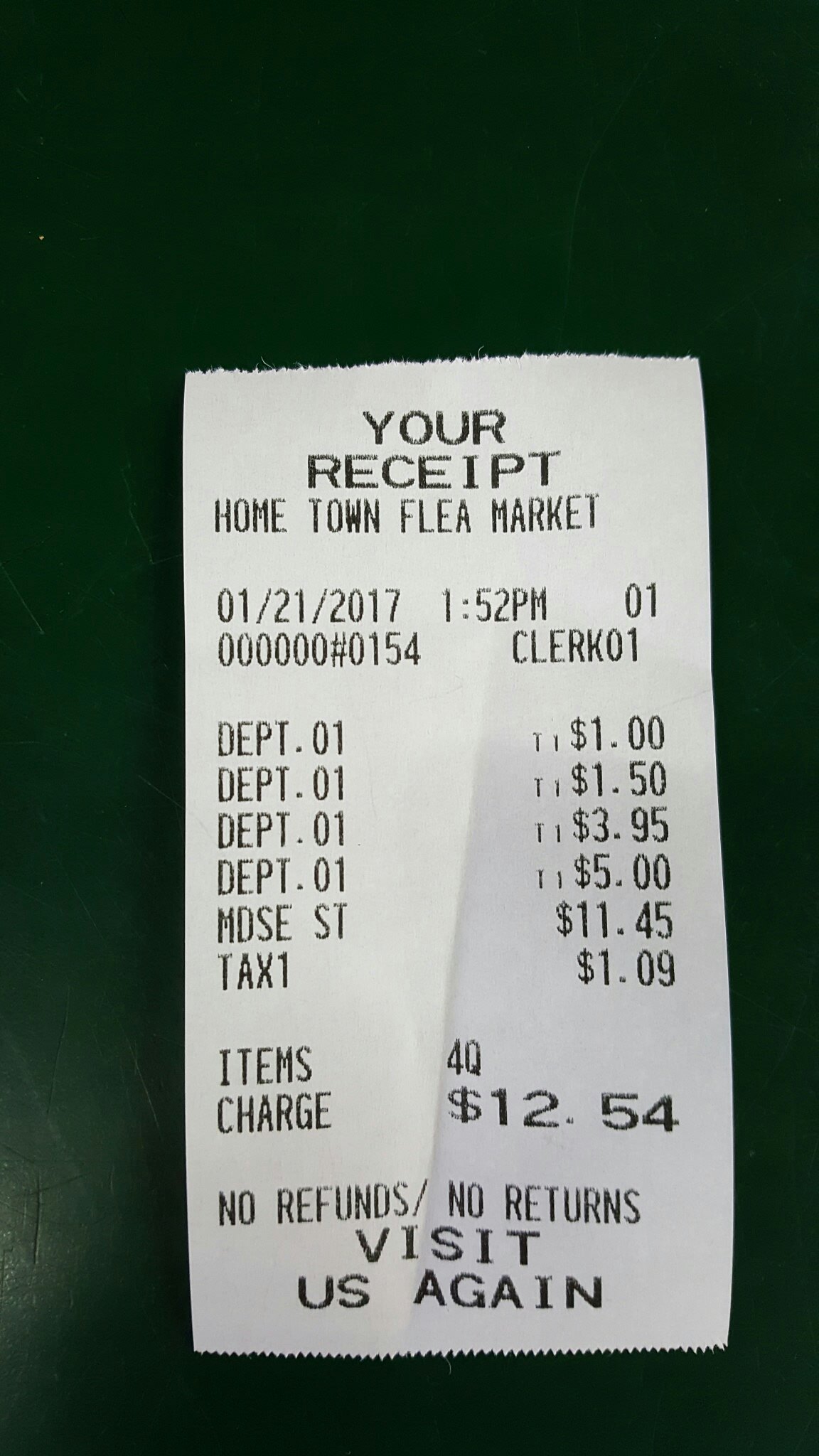The image features a detailed view of a smaller, white receipt with black, computer-generated text. Positioned centrally on a green background, the receipt prominently displays the heading "Your Receipt" at the top, followed by "Your Hometown Flea Market," all in capital letters. It is dated 01-21-2017 at 1:52 p.m. The clerk and department are both identified as "01," repeated multiple times to indicate various transactions. The receipt lists four items coded under Department 01, showing distinct prices: $1.00, $1.50, $3.95, and $5.00. Additionally, there is a merchandise item entry "MDSEST" priced at $11.45 and a tax listed as $1.09. The total charge for the purchase is $12.54. At the bottom, the receipt notes: "No refunds, no returns. Visit us again."